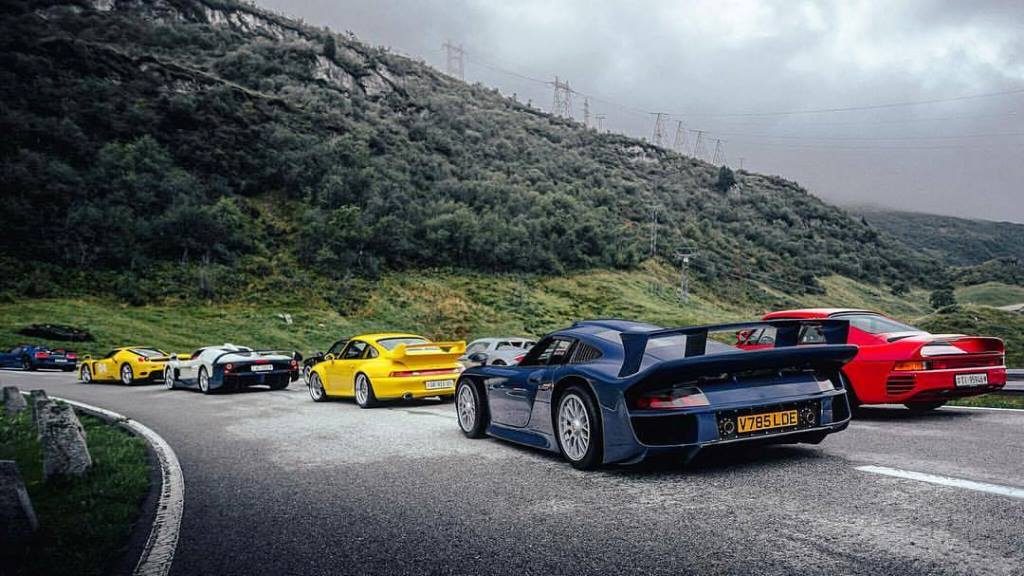In the outdoor image, multiple high-performance and muscle cars are seen racing on a winding two-lane road, which is delineated by dashed white lines in the center and solid white lines on the outer edges. The road curves gently to the left. The prominent cars in the scene include a blue sports car with a matching blue spoiler and a yellow license plate reading "V 785 LDE," a red sports car with a spoiler and an unreadable white license plate, a yellow Porsche-like vehicle with a spoiler, and a gray car. In total, there are approximately a dozen cars visible, suggesting a convoy or race scenario.

The bottom left of the image features a grassy area with scattered rocks, resembling a rudimentary guardrail. Above the road, a large hill covered in trees and bushes stretches across the middle to the upper left portion of the picture. Power lines are visible at the top of the hill. The sky, occupying the top right of the image, is a mix of gray and white clouds, with hints of sunlight attempting to break through. The dominant colors in the image include gray (road and sky), green (grass and trees), and the varied hues of the cars: blue, red, yellow, and gray. The overall setting suggests a highway or a country road rather than a formal racetrack, and the scene captures the cars mid-motion, even though the wheels appear still.